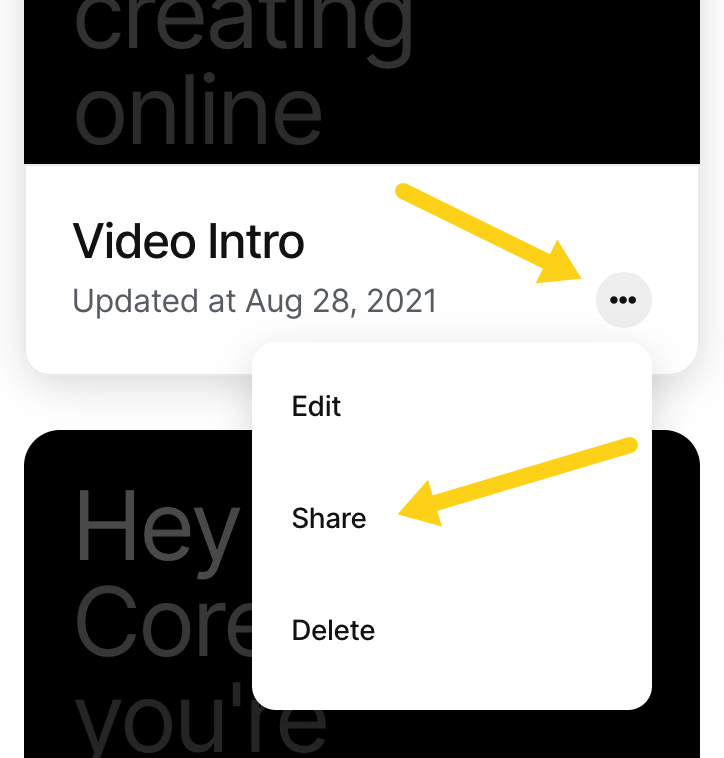This is a detailed caption describing a screenshot of a mobile interface:

---

The screenshot appears to be taken from a mobile device. At the top of the screen, a thick black bar displays the words "Creating Online" stacked in large, light gray letters. Below this bar, a white section displays the text "Video Intro, updated on August 28th, 2021." A large yellow arrow points towards the three vertical dots on the right side of this section, indicating a drop-down menu with options to Edit, Share, and Delete. Another large arrow, oriented right to left, points downward at the word "Share."

Below this, there is a dark gray area with light gray text. The text reads "Hey, C-O-R-E," although the rest of the word following "C-O-R-E" is unclear. Underneath this line, partially visible, is another line starting with "Your" and followed by "Y-O-U-R-P-O-S-T-E-R," but the bottom part of the text is cut off, making the rest of the message unreadable. The interface’s top and bottom sections feature rounded corners and the white area beneath the top bar has a drop shadow. The gray section below does not have a drop shadow.

The screenshot captures a glimpse of an interface related to video content, likely allowing users to share, edit, or delete entries. The visual elements suggest it could be part of an online platform or app designed for creating or managing video introductions.